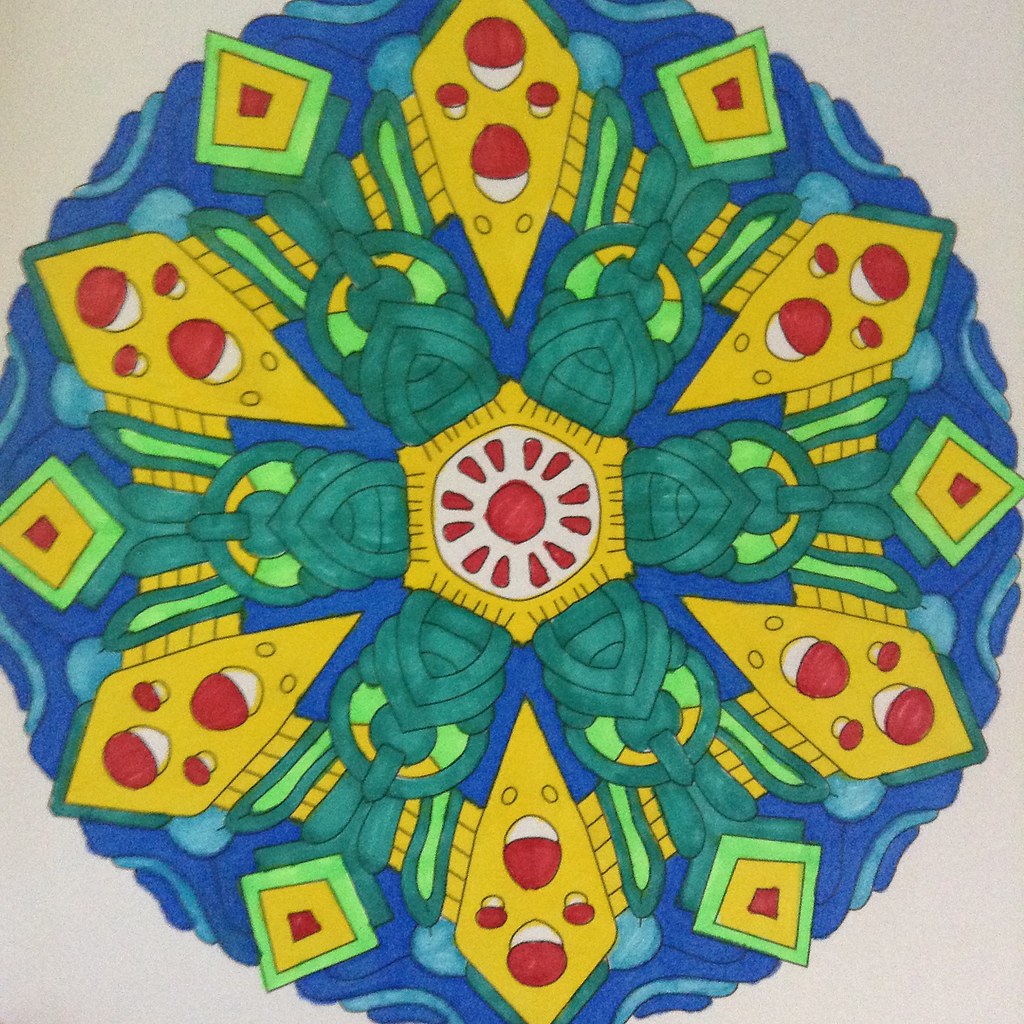This intricate abstract illustration features a multitude of vibrant patterns and shapes rendered in what appears to be watercolor or colored pencil on an off-white, beige square background. At the heart of the image is a central hexagon, solid yellow in color, encasing a white circle with a red dot at its center. Surrounding the dot are red, teardrop-shaped formations, reminiscent of pomegranate seeds or flower petals, radiating outward.

Encircling the central motif, there are six teal, knot-like structures extending from the hexagon's vertices, resembling tied ropes or Hershey’s Kiss shapes. These knots are connected to the outer perimeter of a yellow and black striped hexagon by green, bunny ear-like shapes. Interspersed among these are six yellow, pizza slice-shaped forms, each adorned with abstract red and white mushroom-like designs.

The entire composition sits against a dynamic background of dark blue transitioning to light blue, forming a twisted, wreath-like circular pattern. This kaleidoscopic image is both detailed and symmetrical, presenting a captivating blend of shapes and colors that evoke the sensation of looking through a spirograph or kaleidoscope.